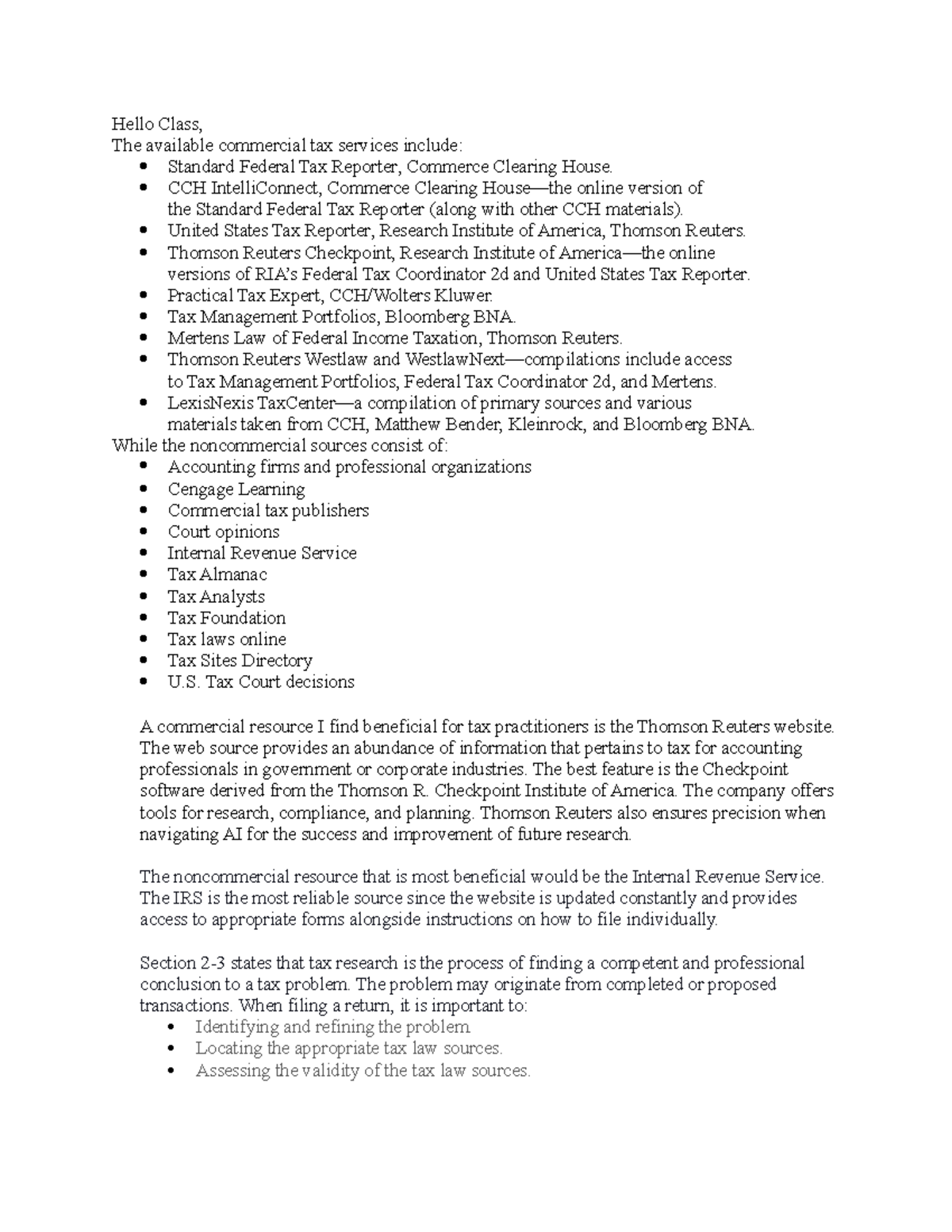**Caption:**

The screenshot, likely from a tablet or mobile phone in portrait mode, depicts a syllabus for a commercial tax preparation class. The background is white with black text. At the top, the header reads, "Hello, class, the available commercial tax services include." This is followed by a comprehensive bulleted list of commercial tax resources:

- Standard Federal Tax Reporter
- Connect Commerce Clearinghouse (online version of the Standard Federal Tax Reporter)
- United States Tax Reporter
- Research Institute
- Thomson Reuters Checkpoint Research Institute
- Practical Tax Expert
- Tax Management Portfolios
- Mercer's Law Federal Income Taxation
- Thomson's Westlaw and Westlaw Next, with access to Tax Management Portfolios

Below this list, there is another set of bulleted points detailing non-commercial sources:

- Accounting firms
- Cengage Learning
- Commercial tax publishers
- Court opinions
- Internal Revenue Service (IRS)

At the bottom, there is a section titled "The commercial resource I find beneficial for tax practitioners," explaining why the Thomson Reuters website is highly recommended. Following it is a brief discussion on non-commercial resources, highlighting the IRS website as the most reliable due to its constant updates.

The final segment touches on "Section 2 to 3," which states that tax research is the process of finding a competent professional conclusion to a tax problem. It includes troubleshooting guidance for potential sources of tax issues. Overall, the document serves as a detailed syllabus for students preparing to become commercial tax accountants.